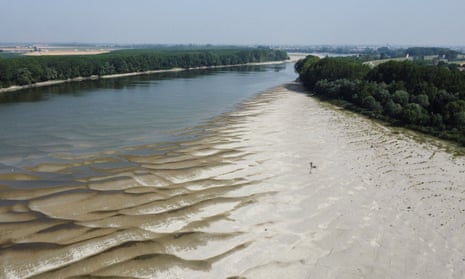This image is a photograph capturing a serene river area, possibly resembling the Mississippi River, flowing into a delta. On the left side of the image, the river is bordered by a shoreline densely populated with shrubs and trees. To the right, closer to the camera, there's another section of shore, similarly lined with trees, and extending into a sandy area. The water itself is slightly blue but transitions to a more brownish hue as it reflects the bright light. The horizon features yellowish patches of ground under a hazy, light blue sky, giving a sense of depth. Towards the foreground, there appears to be an object in the water, potentially a duck, though the scale makes it ambiguous—it could also be a buoy or a small boat. Light reflections on the water's surface add to the tranquil ambiance of this landscape snapshot.